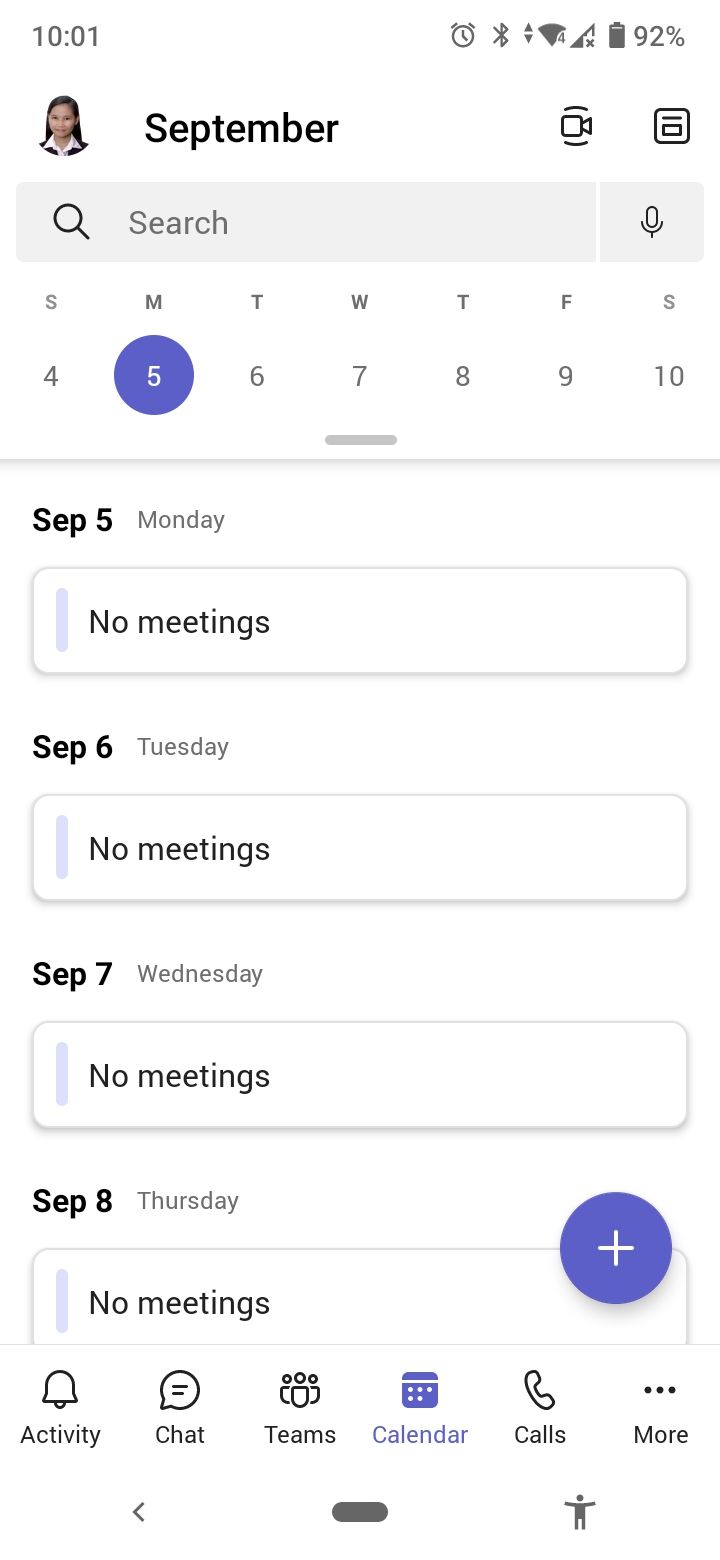This is a detailed screenshot of an Android device showing the user's calendar on Monday, September 5th at 10:01 a.m. At the top-right corner of the screen, an alarm clock icon is visible beside the battery icon indicating a 92% charge, and the Wi-Fi icon. Below the status bar, the user's profile photo appears on the left in a circular icon, followed by the month "September" in text, and to its right, a camera icon likely used to either set up or start a meeting. A search bar with a gray microphone and magnifying glass icon is positioned below the month header.

The calendar is displayed in a classic format, starting with a row of single letters representing the days of the week: S, M, T, W, T, F, S. The current date, September 5th, is highlighted with a purple circle, and to its left, Sunday the 4th is displayed. Beneath the days of the week, the dates are shown in a slightly larger font, including 4, 5, 6, 7, 8, 9, and 10.

A section divider separates the date row from the event listings below. It shows "September 5th, Monday, no meetings," followed by entries for subsequent days: "September 6th, Tuesday, no meetings," "September 7th, Wednesday, no meetings," and similarly, no meetings listed for Thursday. At the bottom of the screen, there's a prominent purple plus icon within a circle, likely used for adding new events or tasks.